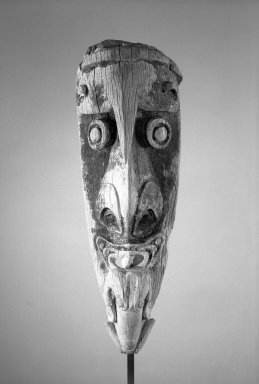This black and white photograph features an elongated, humanoid African tribal mask mounted on a black pole. The mask is crafted from weathered wood, hinting at its age and historic significance. At the top of the mask, a fringe or top of the skull is visible, possibly suggesting hair. A central horn protrudes from the forehead, flanked by decorative imagery on each side. The mask has round eyes with distinct, round pupils and shows a beak-like nose with visible nostrils. Below the nose, a mouth reveals some teeth, giving the mask a somewhat menacing expression. Beneath the mask's mouth is a part that resembles a beard, followed by an arrow-like structure that transitions into the holding pole. The background consists of textured shades of white, black, and gray, accentuating the intricate details and evocative features of this ancient artifact.